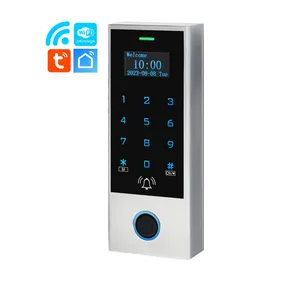This photograph features a white and black device centrally placed, with various logos indicative of Wi-Fi signals apparent in the top left corner. The primarily white and black rectangular device, taller than it is wide, showcases a small digital screen at the top displaying "welcome 10:00" along with other digits "20230648." Below the screen, the device features a keypad with glowing blue buttons numbered 1 through 9, including the pound (#) and asterisk (*) keys. At the very bottom, a distinctive round button, highlighted with a blue outline, sits against a white background, accompanied by an illustration of a ringing bell. This likely suggests that the device functions as both a keypad for unlocking a door and a doorbell, enabling entry through a numerical code and providing a doorbell feature when the bottom button is pressed.